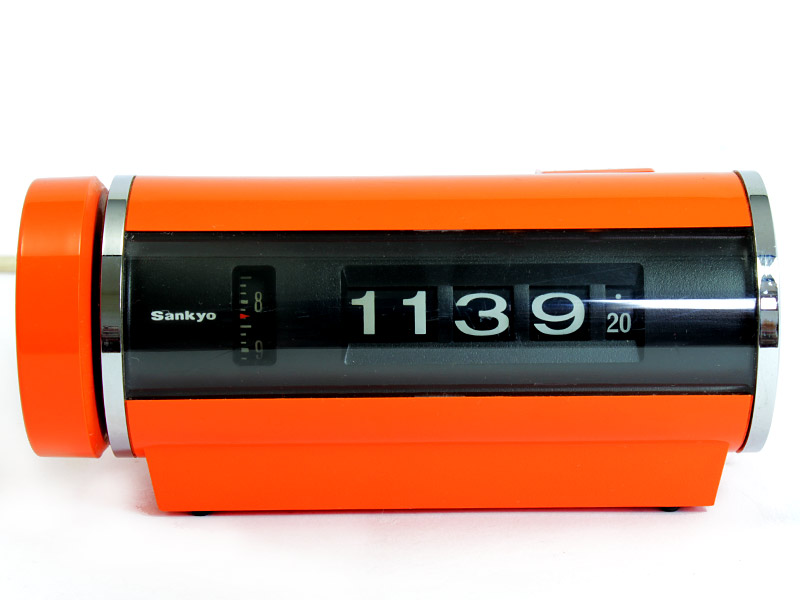This photograph depicts a uniquely designed alarm clock resembling the shape of a battery lying on its side. The clock features a predominantly orange body with a central black section. The brand name "Sankyo" is prominently displayed in white letters on the left side. Adjacent to the brand name, there is a small vertical box with indistinct numbers, and next to it, a larger rectangular display shows the time, "11:39," and "20" in white numerals. The top section of the clock is also orange, while the right side includes a band of silver at both the top and bottom, adding a metallic accent to the overall design. The distinct appearance and unusual battery-like form make this alarm clock a striking and unconventional timepiece.